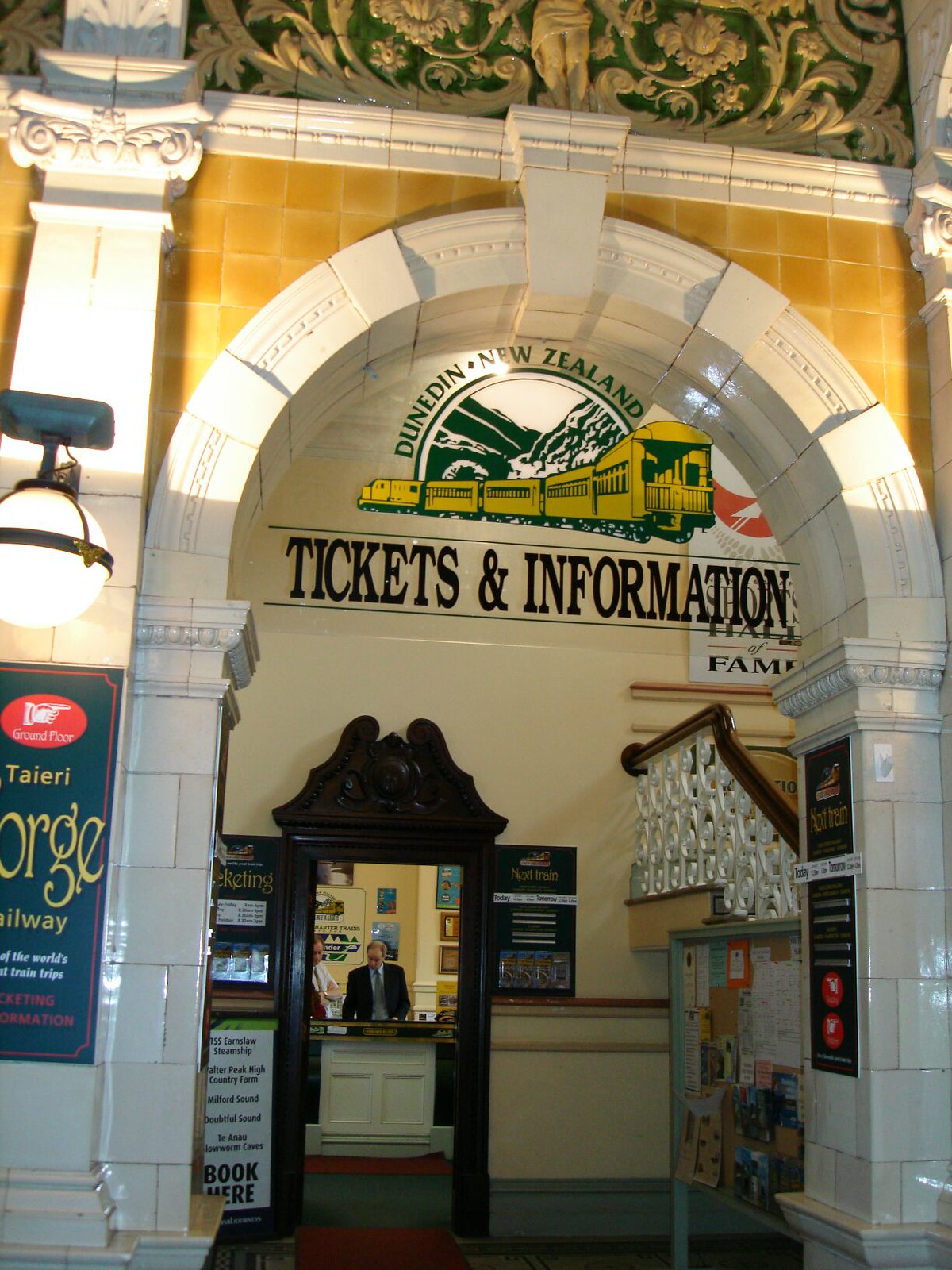The photograph captures the grand entranceway of a historic train station's ticket and information building in Dunedin, New Zealand. Dominating the scene is an imposing arched doorway, vividly illuminated by an ornate globe light on the left side. Above the arch, bold letters spell out "Tickets and Information," surmounted by a symbol of a freight train and the text "Dunedin, New Zealand."

Inside, a smaller arched opening houses a well-dressed assistant, standing behind a wooden counter that serves as a ticket podium. This area is cozy and framed by intricate wooden carvings that resemble an eagle or a shield. The assistant's professional demeanor adds a touch of formality to the old-fashioned charm of the setting, which also features a beautifully ornate wooden handrail leading up to an upper floor. To the left of the assistant, a sign reads "Book Here," inviting travelers to secure their tickets. The photograph captures the intricate blend of architectural elegance and practical functionality at the heart of this historic train station.